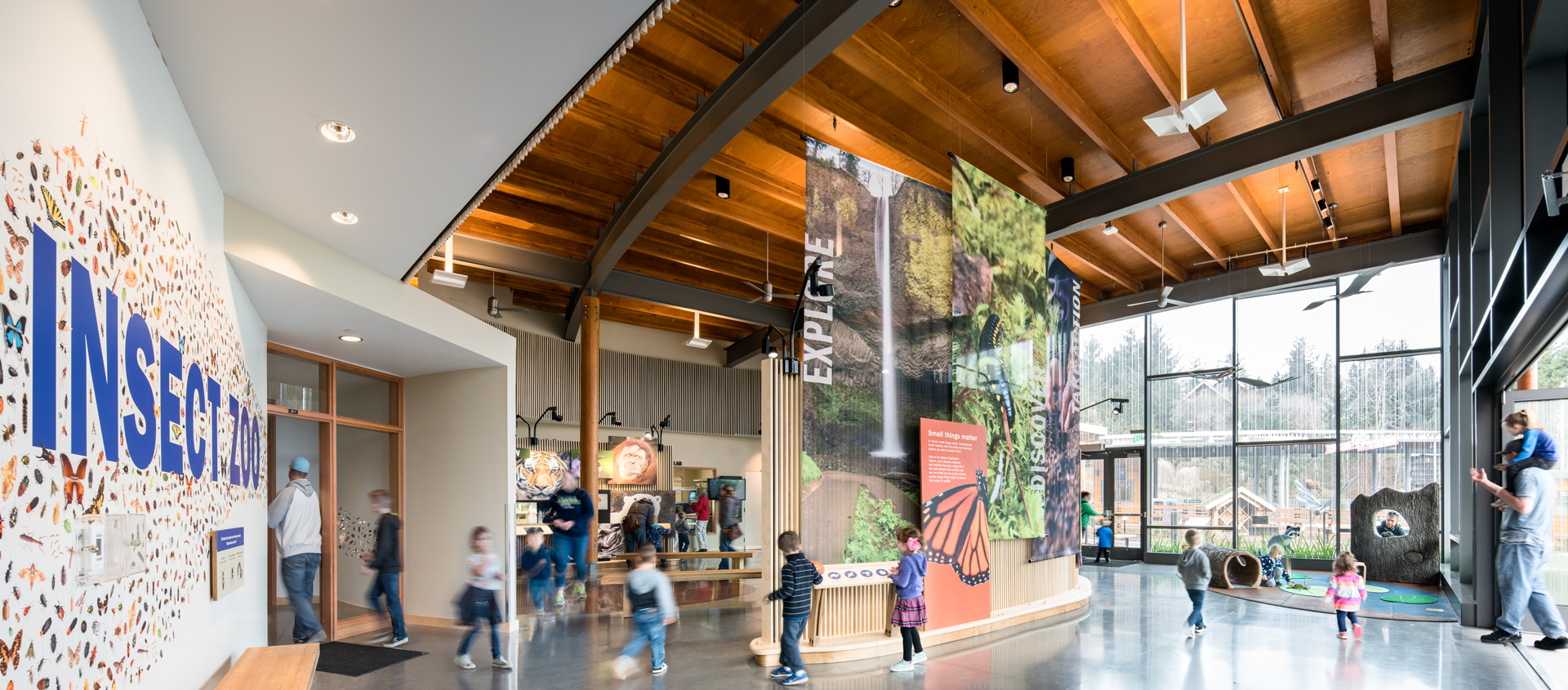This is a detailed photo of the entryway to a vibrant and inviting Insect Zoo, possibly located within a science or children's museum. The modern architecture features a striking combination of wood and glass, with high ceilings made of wood that accentuate the spaciousness of the area. The entrance is primarily composed of an expansive glass wall and door, through which a bustling scene of families can be observed.

Inside, the zoo greets visitors with a large wooden structure in the center, adorned with towering posters depicting various parts of the exhibit, each approximately 10 feet tall. These informative and visually appealing posters guide guests on what to expect as they venture further. The left wall prominently displays the words "Insect Zoo" in a bright blue color, surrounded by an array of detailed insect illustrations, including butterflies and other species, reflecting the educational essence of the venue.

Children and adults alike populate the space, with numerous kids running around excitedly, exploring their surroundings. The casual attire of the visitors, with no heavy jackets, hints at a mild, enjoyable day. Nearby, a store can be glimpsed, adding to the amenities available for a fun family outing.

Overall, the clean, contemporary design, coupled with the engaging and colorful displays, makes this insect zoo an attractive destination for families, especially with young children eager to learn about nature and the fascinating world of insects.